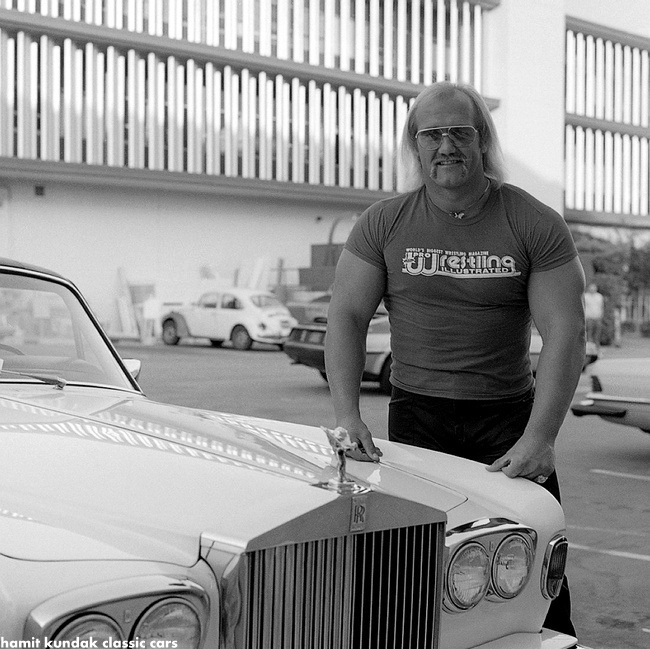The black-and-white photo captures a younger Hulk Hogan standing in a parking lot, smiling and dressed in black pants and a white short-sleeved shirt emblazoned with "Pro Wrestling Illustrated" in white letters. Hulk Hogan, donning sunglasses, has his hands on the long white hood of a Rolls Royce, prominently displaying the iconic grill, lights, and hood ornament. In the background, several classic cars, including an old Volkswagen Beetle and what appears to be the back half of a Mercedes SL, are visible against the backdrop of a large building with a white concrete foundation and rows of windows. A sports car resembling a DeLorean drives through the scene. The parking lot is marked with white stripes for parking spaces, and at the bottom left-hand corner of the image, the text "Hammett, Kondak, Classic Cars" is visible. The photo, bright and clear due to natural light, focuses solely on Hulk Hogan and his striking Rolls Royce, emphasizing the vintage ambiance and automotive elegance of the setting.